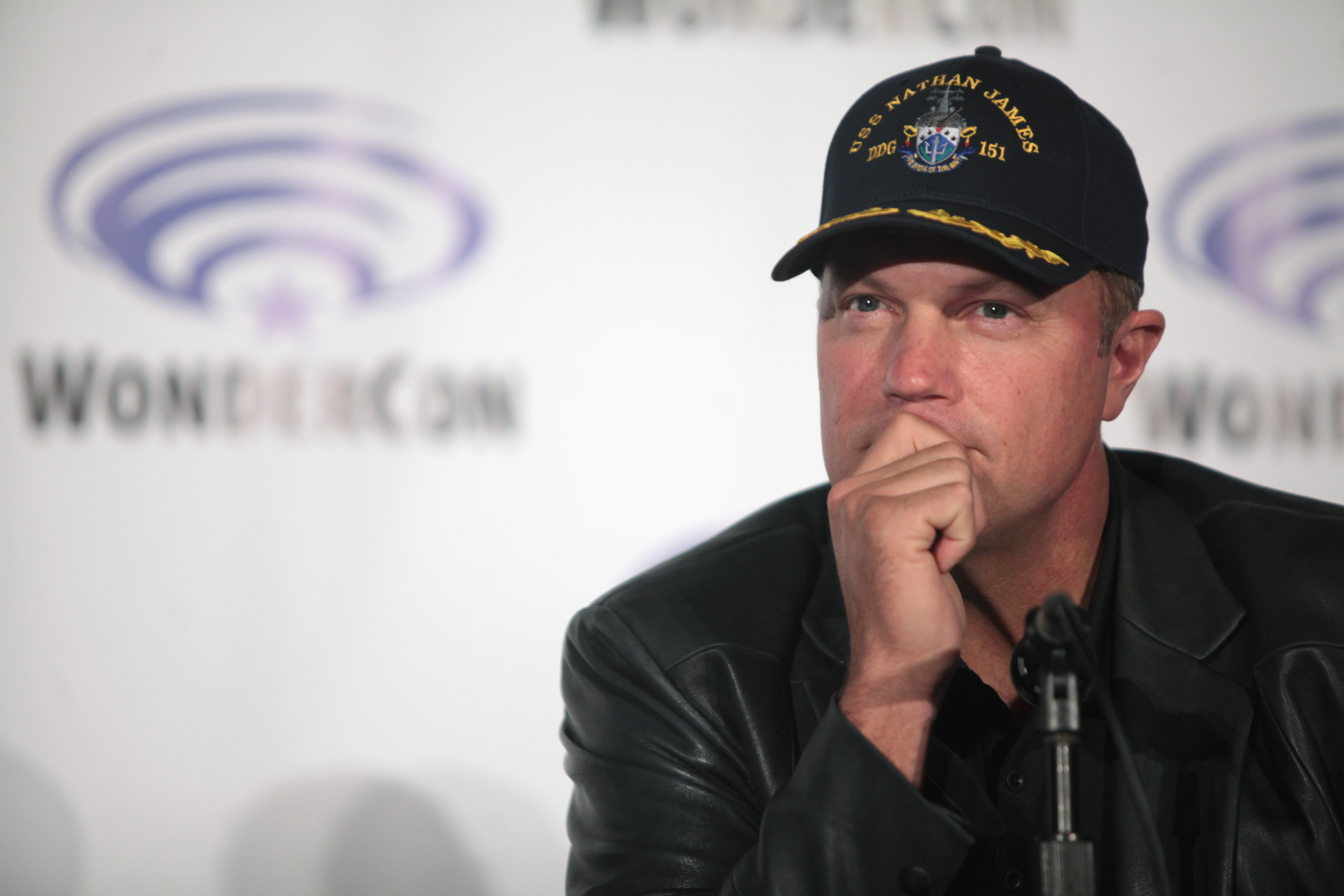The photograph captures a middle-aged white male, likely in his 40s or 50s, sitting at a panel during WonderCon, identifiable by the white banner with a blue spiral star logo behind him. He is wearing a black baseball cap that reads "USS Nathan James DDG-151" adorned with military embellishments and a logo of a ship and shield. His attire includes a black leather jacket over a black button-down shirt. The man has blue eyes and is looking slightly to his left, with his hand resting on his mouth in a thoughtful pose. In front of him is a black microphone, although he is not currently speaking.